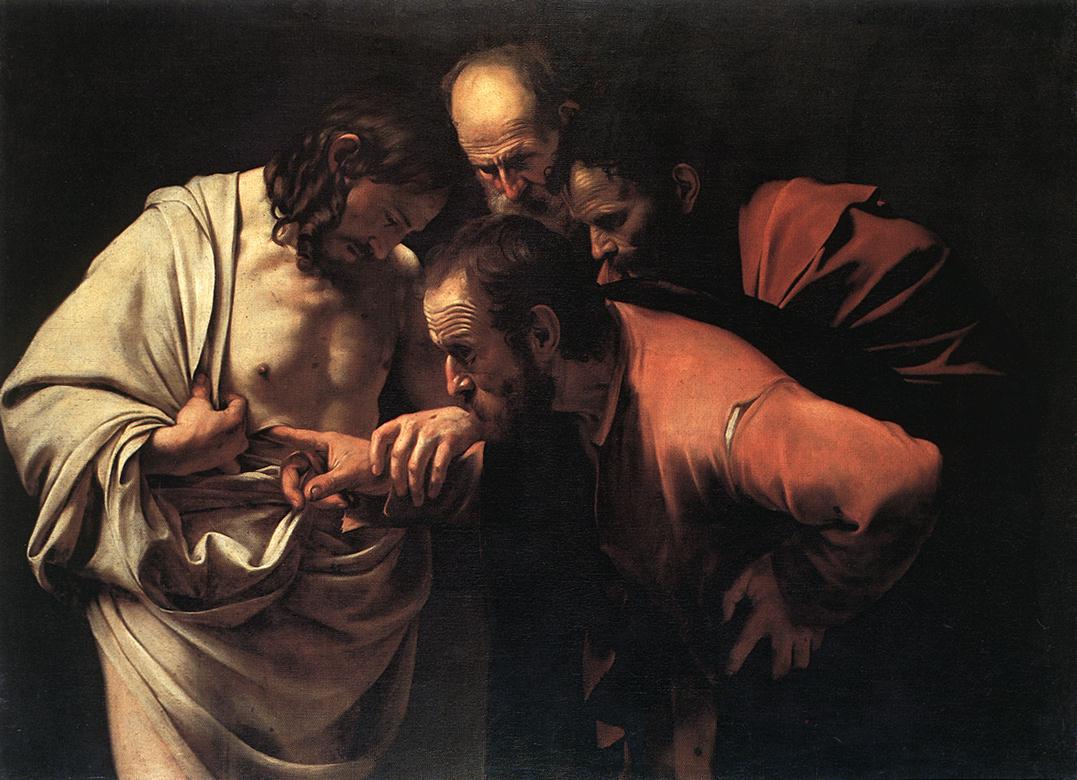The image is a horizontally aligned, rectangular photograph of a painting, which is entirely captured within the photograph. The scene, evocative of the Baroque period, features four men, one of whom is presumably Jesus Christ. Jesus stands on the left, with most of his chest exposed, dressed in a white sheet that he holds back with his right arm. His dark brown, somewhat curly, wavy hair, and his mustache and beard are illuminated by a light shining from the right. Notably, Jesus has a wound, likely from a spear, on his left lower chest beneath the nipple, into which one of the other men inserts his finger.

The three men on Jesus' right are closely huddled together, all intently focusing on the wound. The man directly next to Jesus has a pronounced receding hairline, grey hair, and a grey mustache, with his head tilted downwards, possibly in contemplation. To his right, there is a man with darker skin and dark black curly hair, whose ear and the side of his face are visible as he looks down in concentration. He wears a red cloak with a flowing black collar. The man in the foreground center has long sideburns attached to a beard, wavy brown hair, and distinct ridges above his eyebrows. He appears to be kissing the hand of the man who is touching Jesus' wound, adorned in a dark orange collared shirt with a ruffled front.

The entire scene is set against a pitch-black background, emphasizing the group and their interactions. The painting likely depicts a biblical scene, possibly from the 1400s or 1500s, and resonates with themes from European or Middle Eastern art traditions.